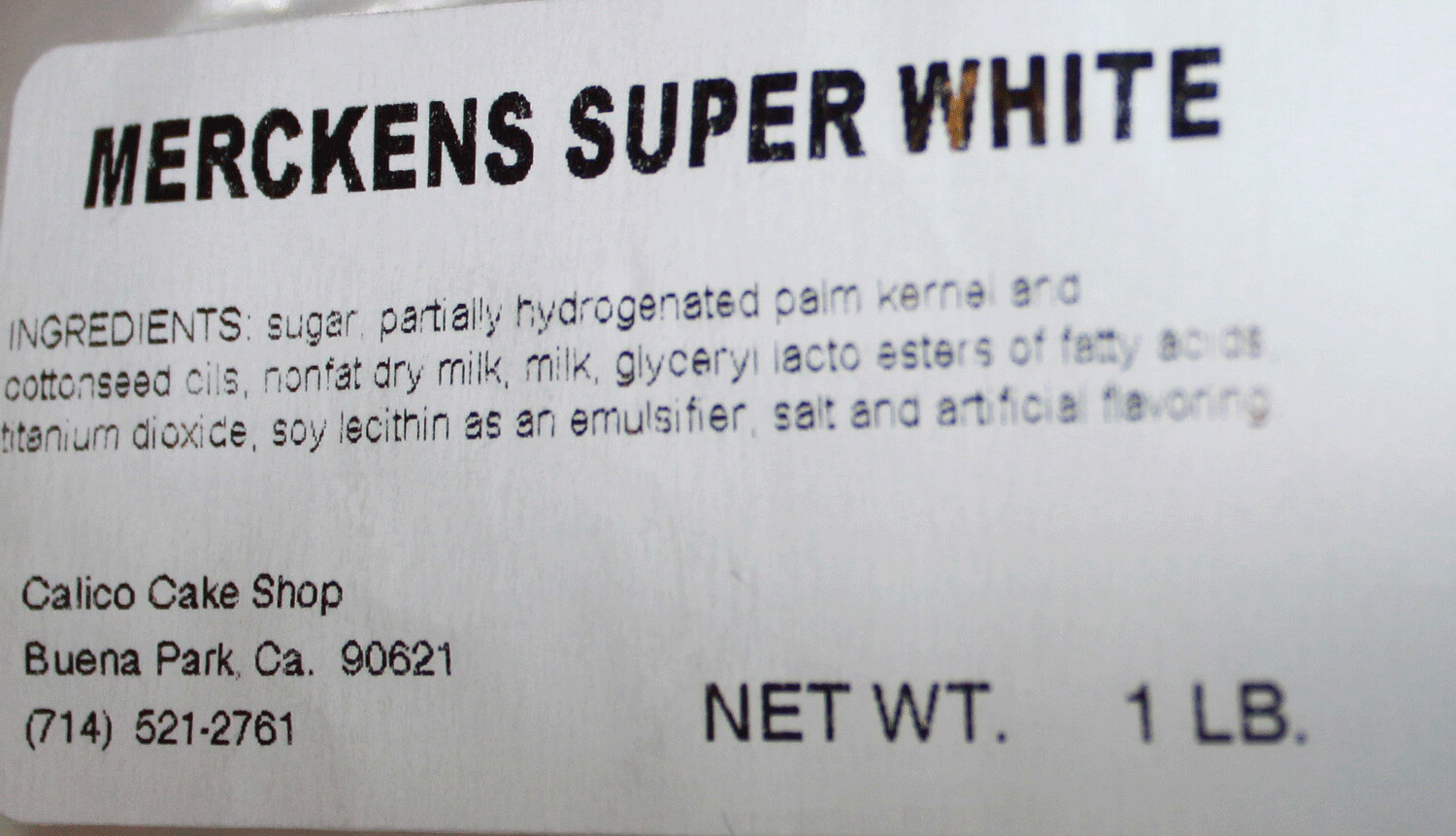This is a detailed, color photograph of an ingredients label from a product. The white label features bold black text at the top that reads "Merckens, Super White." The ingredients listed are sugar, partially hydrogenated palm kernel and cottonseed oils, nonfat dry milk, milk, glycerol lactoesters of fatty acids, titanium dioxide, soy lecithin as an emulsifier, salt, and artificial flavoring. At the bottom of the label, it states "Calico Cake Shop, Buena Park, California, 90621," along with the contact phone number "714-521-2761." The net weight of the product is one pound. The image is an extreme close-up, providing no additional context outside of the label’s borders, with only a hint of the bag visible in the background.